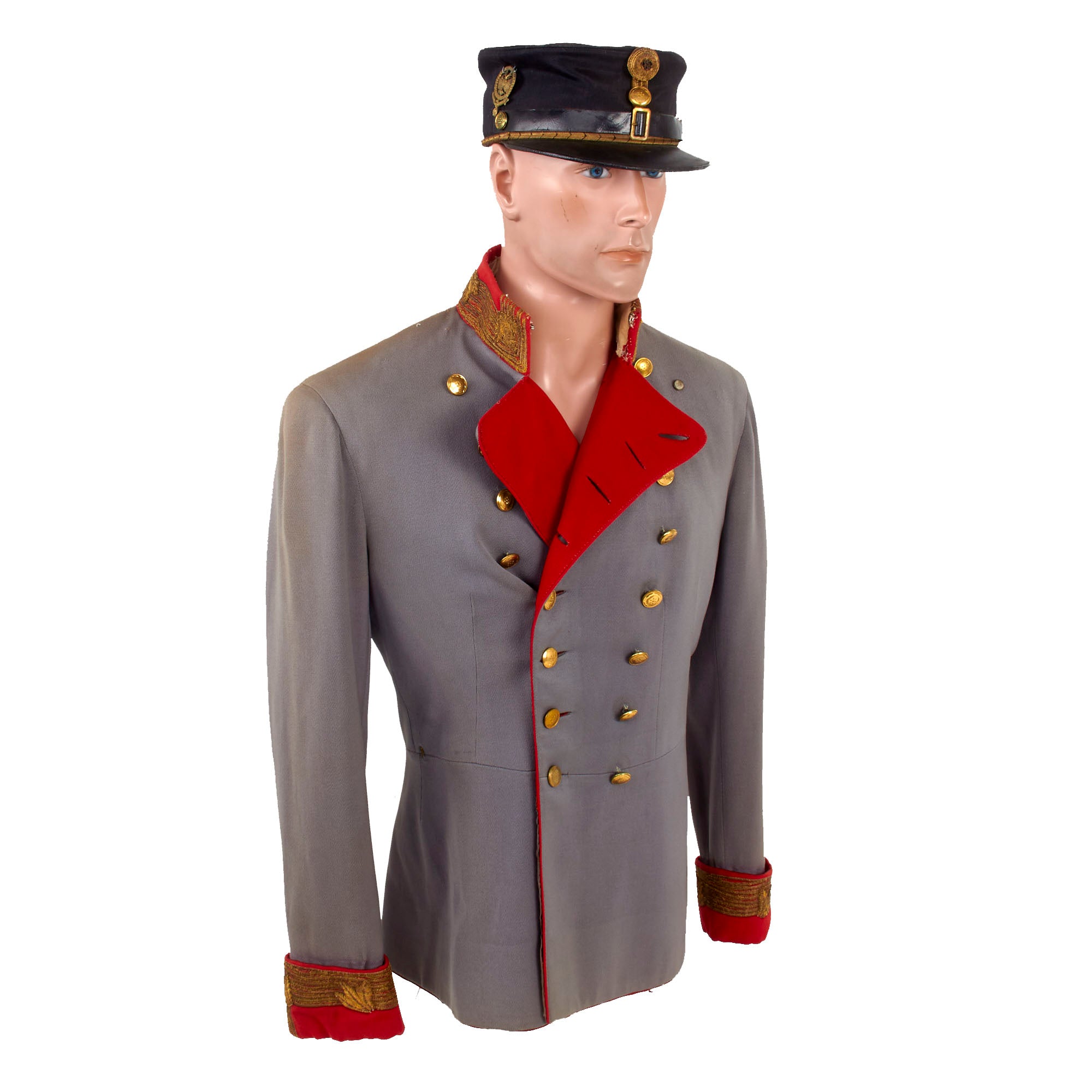The image depicts a pale-skinned mannequin with blue eyes, dressed in an ornate military uniform reminiscent of World War I attire. The mannequin, appearing male, is adorned with a grey jacket featuring a prominent red and gold collar. The jacket's cuffs are red, detailed with gold thread and a leaf-like design. It has two rows of paired gold buttons running down the front. The mannequin is also sporting a black military-style cap embellished with gold accents, including a gold buckle, badges, and gold lining. The overall appearance is meticulously detailed, with the mannequin staring straight ahead, creating a striking and regal soldier-like presence.